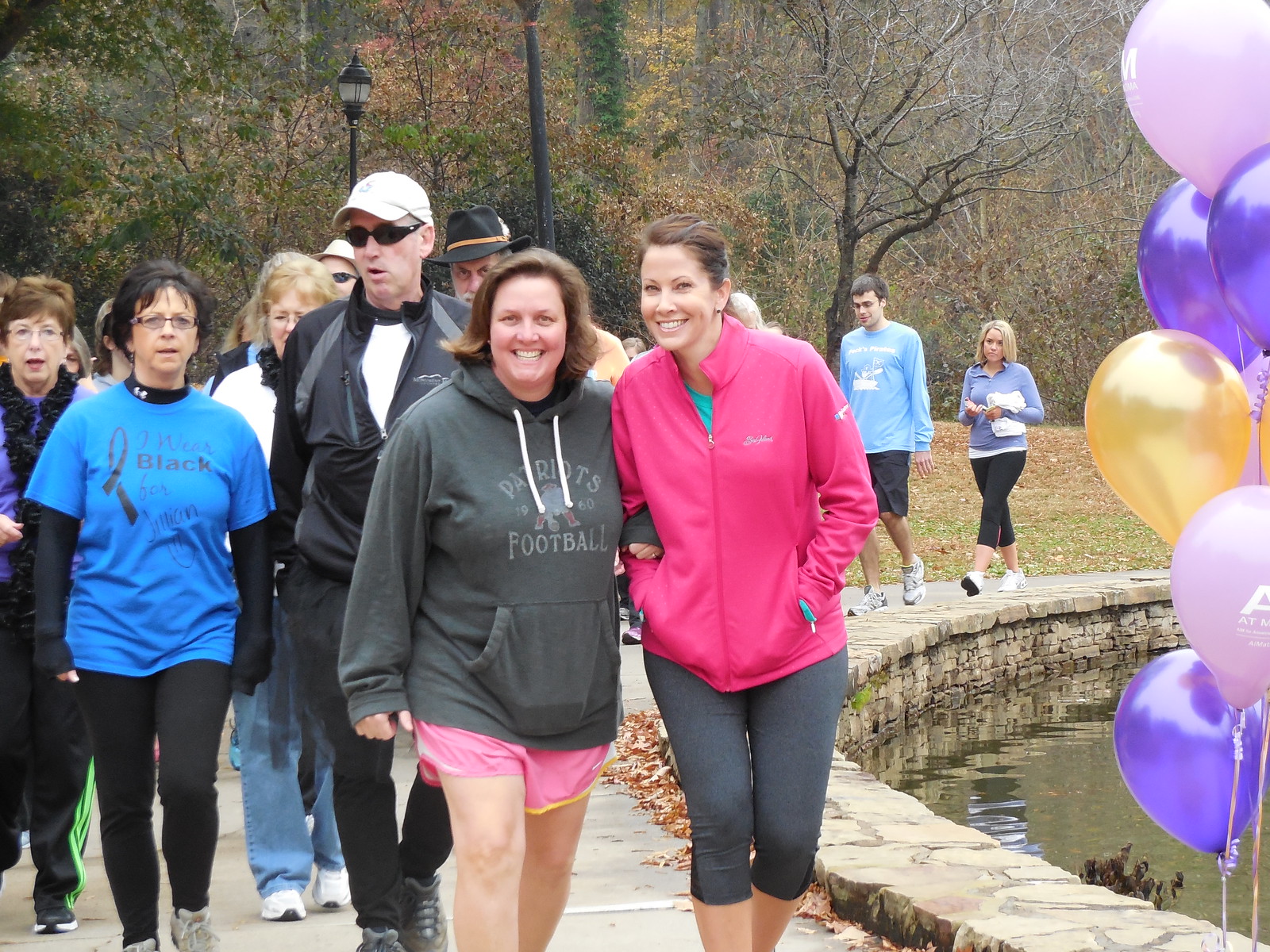A group of people is walking along a paved path encircling a pond with greenish water, which is bordered by a stone wall. Numerous helium balloons in shades of purple, yellow, and pink float along the right side, tethered by white strings to something unseen. The balloons bear some writing, with one displaying the letter "A." The scene appears to be set in autumn, indicated by trees with orange leaves and patches of dying grass in the background.

In the foreground, two women in their 30s lead the group. The woman on the left has light brown hair framing her smiling face and wears a long gray hoodie with white tie cords and white letters spelling "Patriots football." She pairs it with light pink shorts. To her right, another woman wears a pink jacket over a zippered turquoise shirt and gray pants. She's walking arm-in-arm with the first woman.

Behind this pair, several other walkers follow. Among them are three men and several women, some dressed in t-shirts and fleeces, others in long pants and sneakers. A man in a black outfit and white hat walks behind the leading pair, and nearby, a woman dressed in black leggings, a black long-sleeve shirt, and a blue t-shirt that reads "I wear black for Jillian" is easily noticeable. The group appears to be on a casual walk or a hike around this tranquil pond setting.